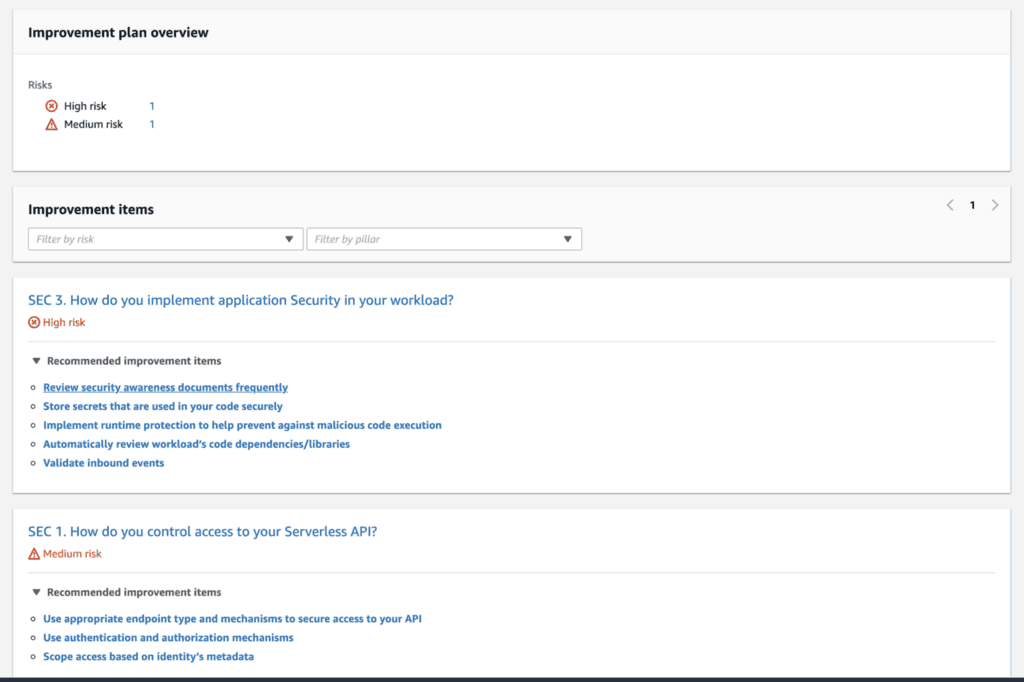The screenshot displays the "Improvement Plan Overview," categorizing risks into "High Risk" and "Medium Risk," each marked by a blue indicator. Underneath this section, there is a list of "Improvement Items," navigable through right and left arrows. The items can be filtered by "Risk" and by the "PILLAR" (P-I-L-L-A-R) category, specifically focusing on "SEC" (S-E-C).

Highlighted within the "High Risk" section, indicated by a red circle with an "X," the recommended improvement item is to "Review Security Awareness Documents Frequently," written in blue. Other recommended high-risk improvement actions also listed in blue are:
- "Store Secrets that are used in your code securely."
- "Implement Runtime Protection to Help Prevent Against Malicious Code Execution."
- "Automatically Review Workloads, Code, Dependencies, Libraries, and Validate Inbound Events."

Additionally, a "Medium Risk" item, identified by the code "SEC1" and marked with a red triangle containing a red question mark, poses the question: "How do you control access to your serverless API?" Recommended improvement items are stated below this query.